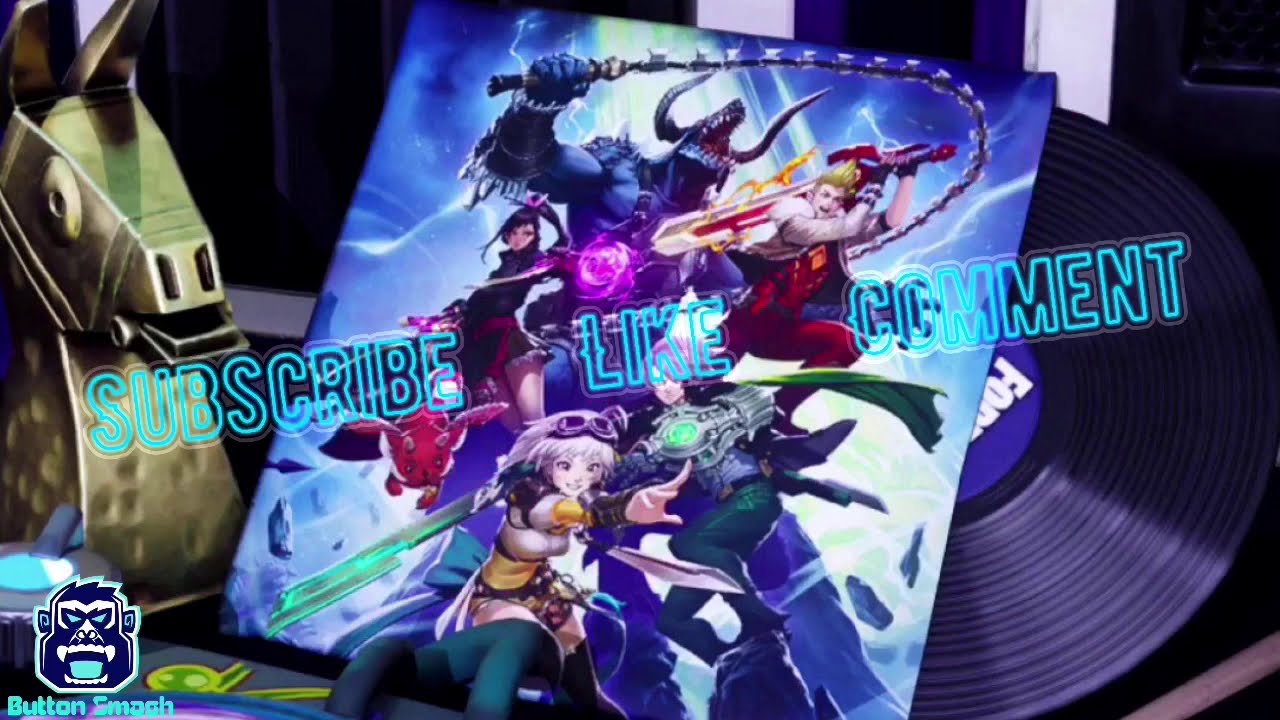The image prominently displays an animated poster, possibly for a video game or comic book, depicting various action-packed characters. Central to the poster is a massive, muscular, blue-skinned beast with horns and a human-like body, gripping a rod. Surrounding this creature are several cartoon characters: a man wielding a large sword with flames, a woman casting a purple ball of magic, and another female character. Additionally, there is a small red creature resembling a fox with dragon features and large ears. Also featured is a tiny red dragon.

In the lower left corner of the image, there is a stylized icon of a glaring monkey head with an open mouth and fangs bared, labeled "button smash" in aqua-colored text. A golden pinata with a unicorn horn appears on the left side of the image, and a record partially emerges from its sleeve labeled "F.O.R.," suggesting a possible Fortnite advertisement. Spread across the image in neon-blue text are the words "subscribe, like, comment."